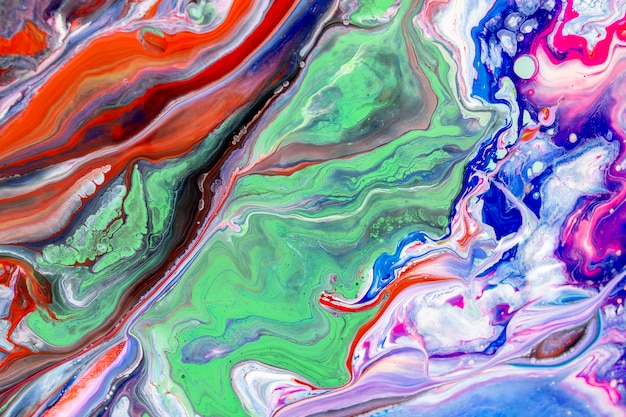The image is a captivating abstract painting that combines a rich spectrum of colors in swirls, streaks, and wavy lines, giving it an impressionistic feel akin to an outer space galaxy or an oil spill. The upper left corner is dominated by bold, wavy lines of reds and whites, creating a dynamic contrast. The middle of the painting, which occupies the majority of the canvas, is filled with vibrant greens and blues that contribute to its depth and complexity. On the upper right and lower corners, the coloration transitions into softer, more mixed hues of pink, blue, white, and a touch of purple, giving the impression of delicate, swirling oil droplets. The entire composition integrates a mesmerizing array of colors—including orange, deep purple, lilac, sea blue, aquamarine, pale blue, gray, and silver—imbued with a light and airy aesthetic on the right side and a heavier, darker palette on the left. The result is an intricate and lively piece that evokes both beauty and mystery.